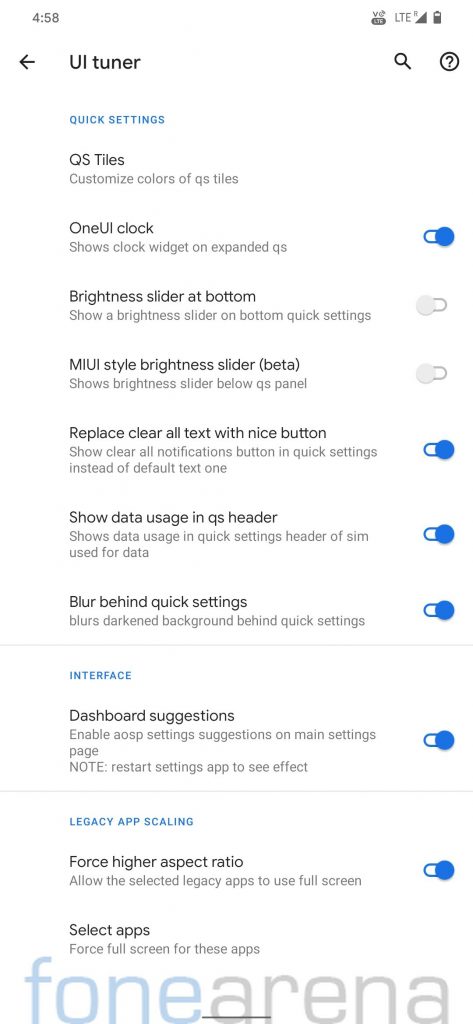The image shows a screenshot from a smartphone displaying a page titled "UI Tuner." At the top, the title "UI Tuner" is in bold black uppercase letters, with a back arrow icon positioned to the left, and search (magnifying glass) and information (black circle with a question mark) icons on the right. The time displayed in the upper-left corner of the screen is 4:58.

Below the "UI Tuner" title, the subtitle "QUICK SETTINGS" is written in uppercase blue letters. This section includes several options:

1. **QS Tiles**: Underneath, a gray description reads "Customize colors of QS tiles."
2. **One UI Clock**: Displays "clock widget on expanded QS." The switch next to it is turned on (blue oval with a solid blue circle on the right).
3. **Brightness Slider at Bottom**: No additional description provided.
4. **MIUI Style Brightness Slider (Beta)**: Indicates it's a beta feature.
5. **Replace Clear All Text with Nice Button**: This switch is turned on (blue).
6. **Show Data Usage in QS Header**: The switch is turned on (blue).
7. **Blur Behind Quick Settings**: The switch is also turned on (blue).

Further down, there is another section titled "INTERFACE":

- **Dashboard Suggestions**: Annotated with "Enable AOSP settings suggestions on main settings page. Note: restart settings app to see effect." The switch is turned on (blue).

The final options include:

- **Legacy App Scaling**: The text is in blue.
- **Force Higher Aspect Ratio**: The switch is turned on (blue).
- **Select Apps**: Displays "phone arena" with "fone" in light blue-gray and "arena" in gray, all in lowercase.

The detailed layout and interactive elements indicate various customizable settings, enhancing the user's interface experience.